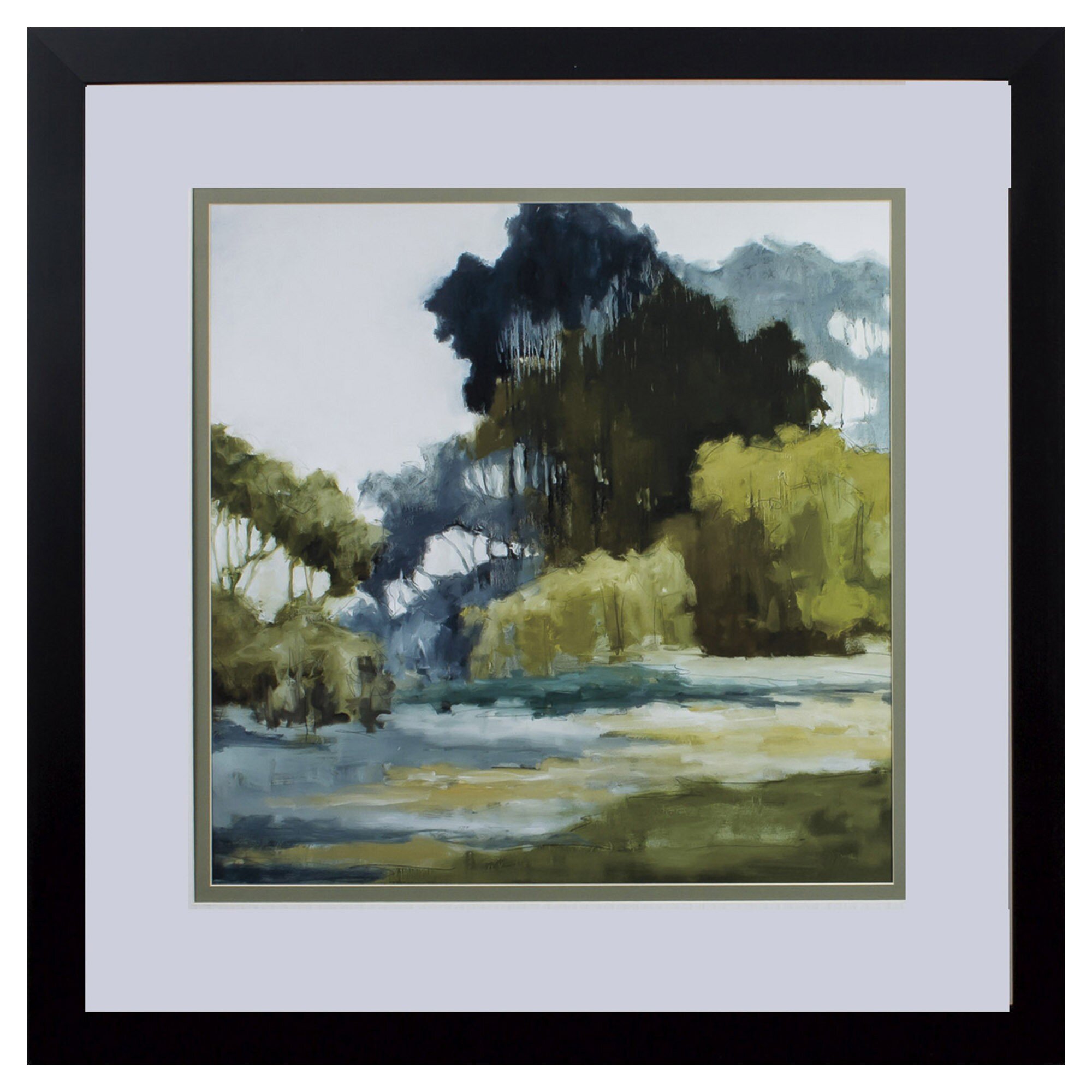This image showcases a painting that is intricately framed. The painting is encased within a thick black picture frame, followed by a substantial white-bordered paper or cardboard frame, which itself is edged by a thin, dark green line. Inside these layers of framing lies the artwork, which has an abstract quality.

The painting features a predominantly white sky in the upper left and right corners, transitioning into a dense canopy of trees. The top tier of trees exhibits a dark green hue, while the layer below is slightly lighter but still quite dark. On the left side, lighter green trees intermingle with smaller trees with hints of gray, creating a varied texture. On the right, lighter green trees are present, along with some blue-toned bushes.

In the middle section of the painting, trees are painted in shades of blue, gray, and various greens, including lime green. Blue trees in the background subtly blend into the scene. A body of water, possibly a creek, runs through the canvas, depicted in shades of blue, green, and yellow. The lower right corner hints at a grassy area.

Overall, the painting, which almost appears to be dripping due to its watercolor effect, lends an ethereal and somewhat moist appearance to the trees and landscape.